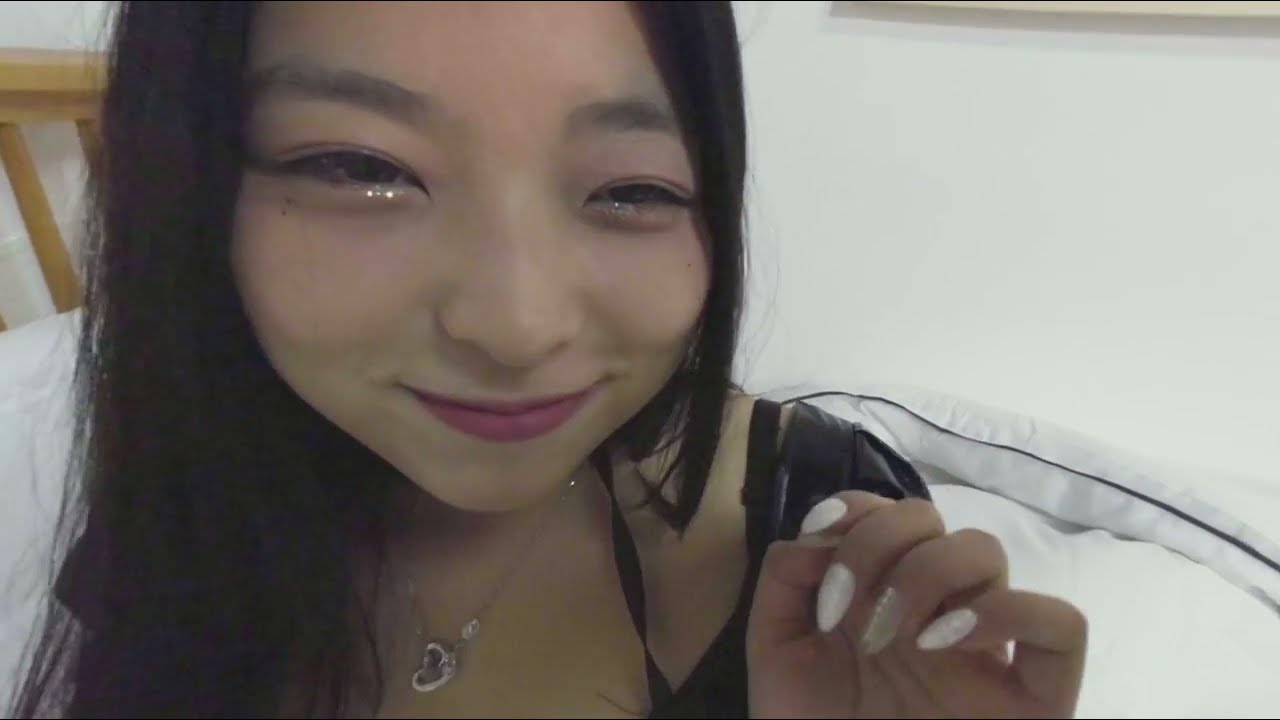The image depicts a close-up of a young Asian woman, likely a teenager, smiling warmly at the camera. She has long, dark hair and is wearing a black shirt, partially visible at her shoulders, along with glitter eyeliner and pinkish-red lipstick. Her accessories include a silver necklace with a heart-shaped pendant. She is holding her left hand up near her left shoulder, showcasing her sharp, pointed fingernails, which are painted white except for a clear polish on the ring finger. She appears to be sitting on a bed, with a white duvet or comforter and a light brown, wicker-style headboard visible behind her. The background includes a white wall. The image shows her face down to just above her chest, although it is slightly distorted, making her face appear wider than normal.